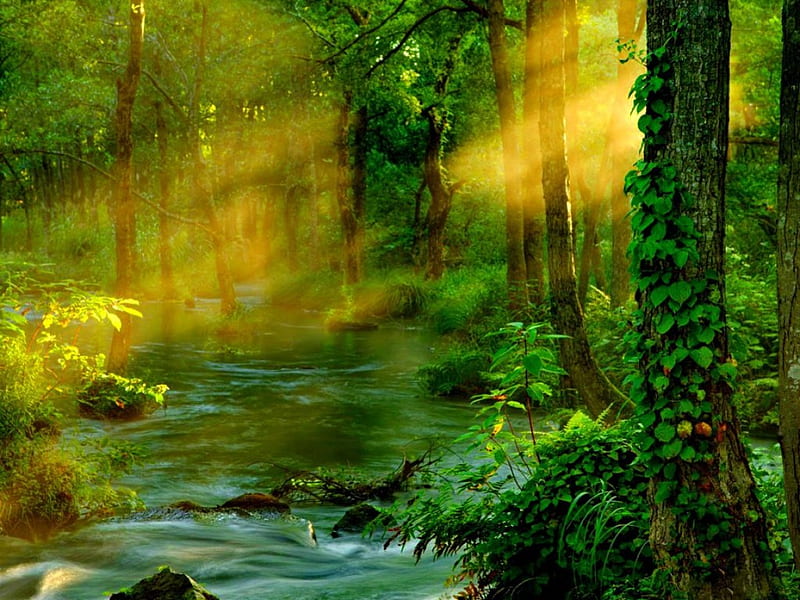In this color photograph of a serene forest scene, a flowing stream cuts diagonally through the center, flanked by lush greenery on both sides. The stream, tinged with teal and white hues, flows over black rocks and is partially bordered by tree trunks and shrubbery on the left. In the background, the dense undergrowth gives way to overgrown green bushes and dark brown tree trunks. On the right, a prominent, grayish-green tree stump stands tall, adorned with green vines and surrounded by plants and bushes. Sunlight streams in from the upper right, casting golden rays that illuminate the peaceful, slightly flooded forest area. Amid the green canopy, the ripples of the water add to the tranquil ambiance, with branches and rocks scattered throughout this seemingly natural, yet slightly manipulated, idyllic woodland scene.